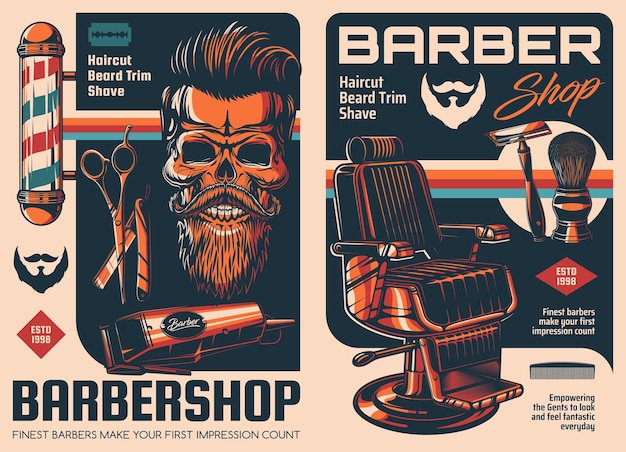This barbershop advertisement is a two-sided masterpiece designed to catch the eye. On the left side, there's a striking image of a skull with a beard, styled into a hipster haircut with a pompadour mustache. The skull, although eyeless, appears to be smiling, adding a touch of whimsical charm. Above this intriguing graphic, the text "Haircut, Beard, Trim, Shave" is prominently displayed, accented with a classic razor blade. Surrounding the skull are various traditional barbershop icons: a red, white, and blue striped barber pole, scissors, a straight razor, an electric razor, a beard, and a mustache. A diamond-shaped graphic declares "Established 1998," anchoring the advertisement in a sense of history. At the bottom of this side, bold lettering announces "Barbershop" followed by the slogan "Finest barbers make your first impression count."

The right side of the advertisement continues the modern yet nostalgic aesthetic with text-heavy graphics. The phrases "Barbershop, Haircut, Beard, Trim, Shave" adorn the top, emphasizing the range of services offered. Below, the tagline, "Finest barbers make your first impression count," is reiterated alongside an additional motivational line, "Empowering the gents to look and feel fantastic every day." This section is visually enriched with images of shaving utensils, including a razor and brush, as well as a traditional barber chair, symbolizing comfort and professional care. This advertisement cleverly blends vintage barbershop elements with a contemporary twist, promising a premium grooming experience.